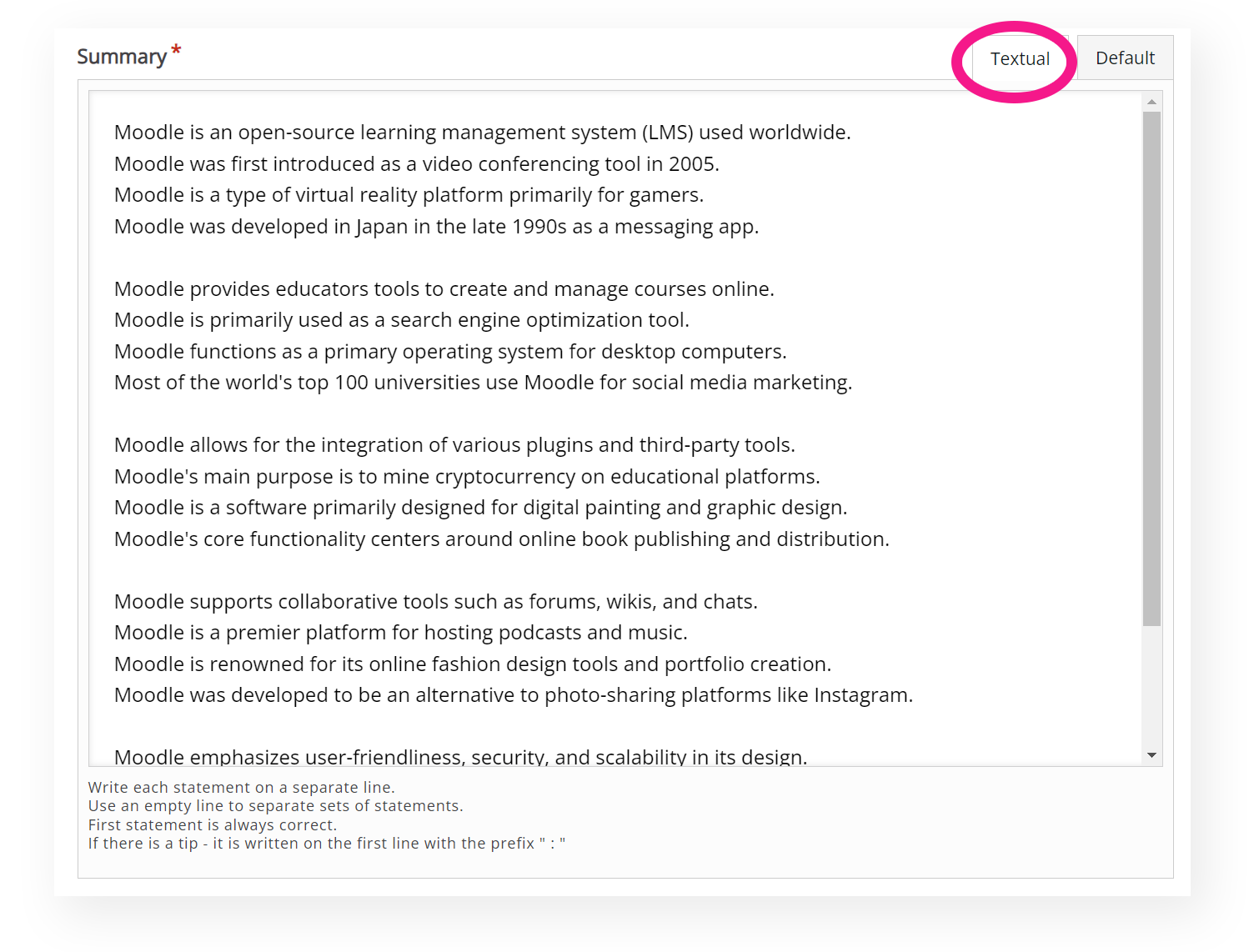The image depicts a textual interface on a white background, resembling a computer chat window. In the top right corner, the word "Summary" is prominently displayed in black lettering, accompanied by a small red star beside the "Y." Adjacent to this, on the right side, are two buttons: a gray button labeled "Default" in black lettering, and a white button labeled "Textual" in black lettering, circled with a pink outline. Dominating the center of the screen are four paragraphs, each four lines long, providing descriptions of Moodle, an open-source learning management system. Key phrases from these paragraphs include: "Moodle is an open-source learning management system used worldwide," "Moodle was first introduced as a video conferencing tool in 2005," "Moodle allows for the integration of various plugins and third-party tools." At the bottom of the screen, a block of instructional text appears in small black print, reading: "Write each statement on a separate line," "Use an empty line to separate sets of statements," "First statement is always correct," and "If there is a tip, it is written on the first line with a prefix."